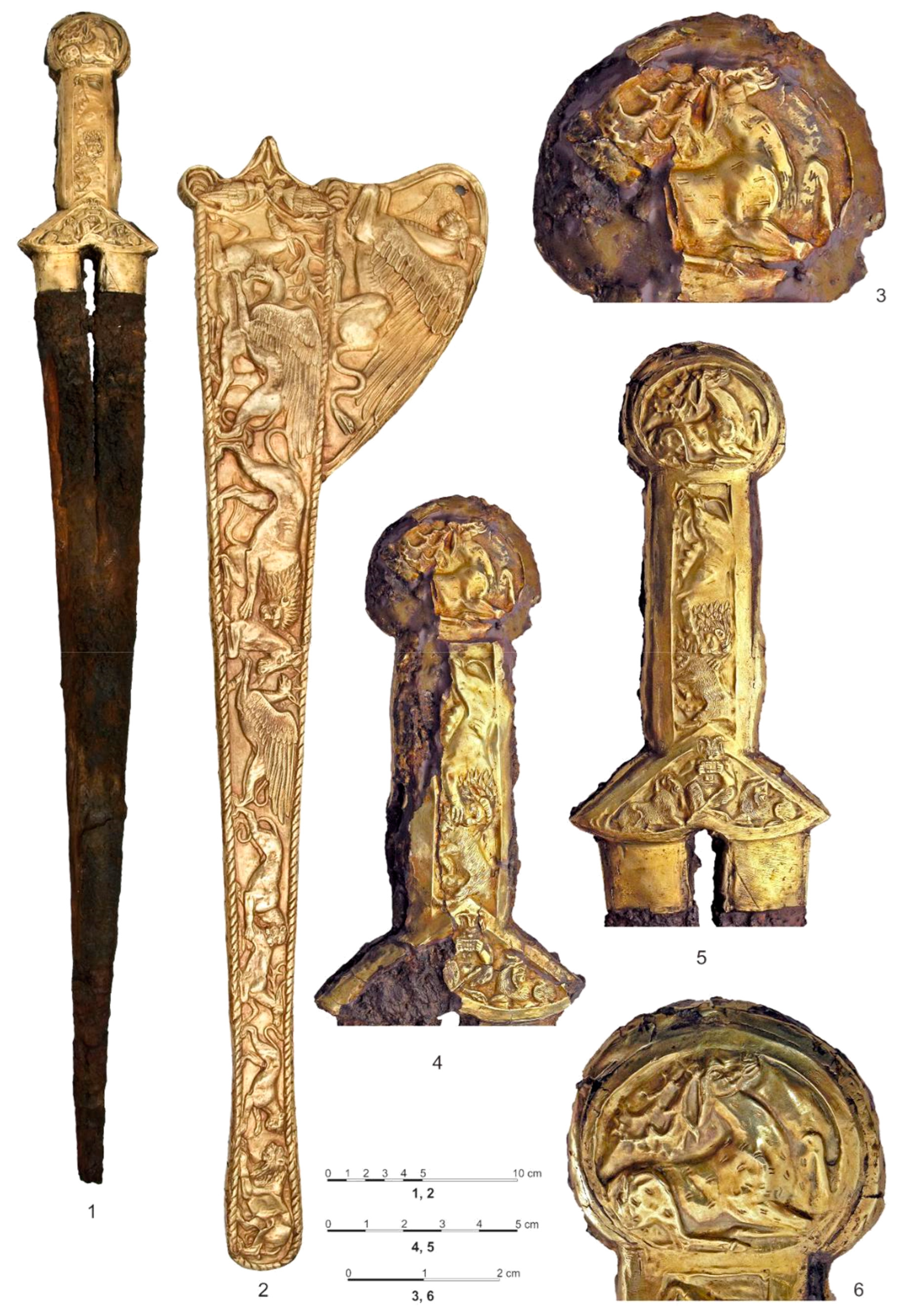This photograph showcases an array of vintage sword and sheath components, meticulously laid out on a white background and labeled with numbers one through six. At the center of the arrangement is a beautifully handcrafted saber, labeled as number one, featuring a handle adorned with intricate gold engravings and hues of gold, copper, and pewter. The blade itself extends into a pointed tip, hinting at its brown metal construction.

Beside the sword, labeled number two, is an ornate sheath. This sheath mirrors the sword's elegance with its detailed engravings of mythical and animal figures, including tigers and winged horses, etched into its gold and copper-colored surface. The sheath's design is both protective and aesthetically aligned with the blade it houses.

Numbers three through six describe various supplementary components of the sword, each contributing to the weapon’s intricate craftsmanship. Number three is a circular gold piece, possibly a pommel or a decorative end cap, featuring detailed etchings of possibly a horse’s head or a person. Both numbers four and five resemble segments that flare out at the bottom, with decorative protrusions and complex designs; number four incorporates notable brown metal elements, while number five, although similar, has longer extensions. Finally, number six is a round disc, etched with a human figure and a horse, surrounded by a darker brown border.

The photograph not only highlights the elegant and ancient artistry of these pieces but also provides a clear legend with measurements at the bottom, emphasizing the detailed and meticulous work put into each component of this vintage sword and sheath ensemble.